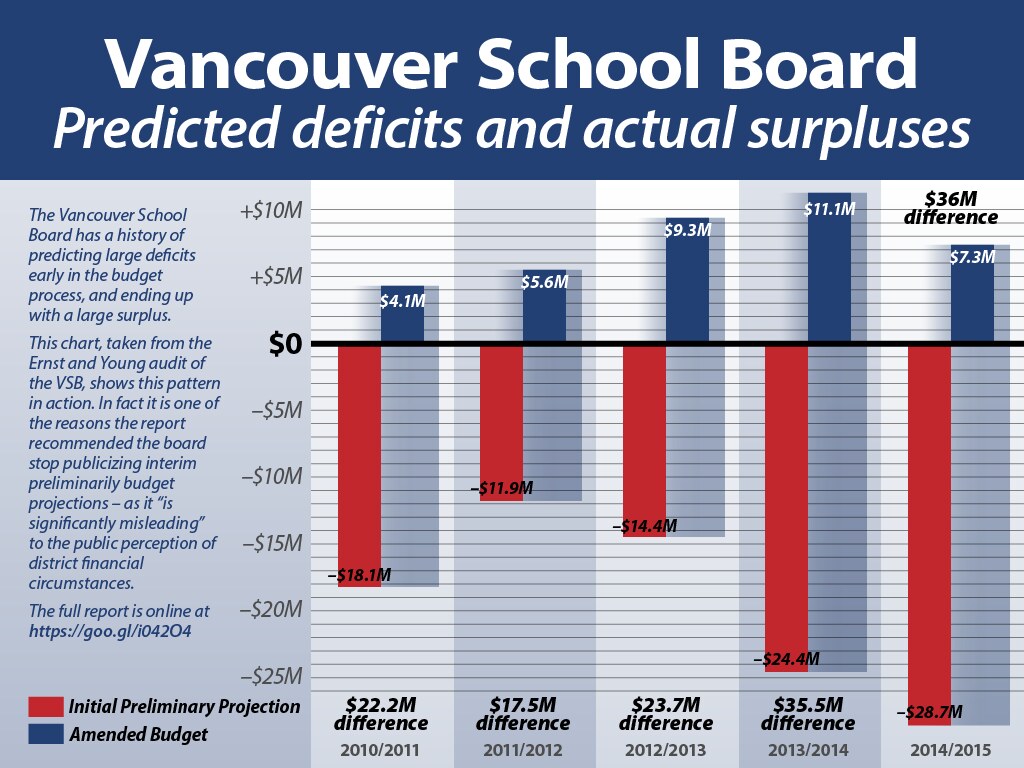The image showcases a detailed bar chart titled "Vancouver School Board Predicted Deficits and Actual Surpluses," with a dark blue banner and white text at the top. This chart is sourced from an Ernst and Young audit and illustrates the Vancouver School Board's historical trend of predicting large deficits, yet consistently achieving substantial surpluses from 2010 through 2015. The left side of the chart states that this pattern has led to recommendations against publicizing preliminary budget projections due to their misleading nature. The graph features five columns, each representing a year, with initial preliminary deficits shown in red (downward bars) and amended budget surpluses in blue (upward bars). The board has managed to convert predicted deficits, ranging from negative $25 million, into surpluses of up to plus $10 million each year, highlighting their impressive financial management. The chart includes extensive text, coding, and values on the bars, contributing to its complexity.